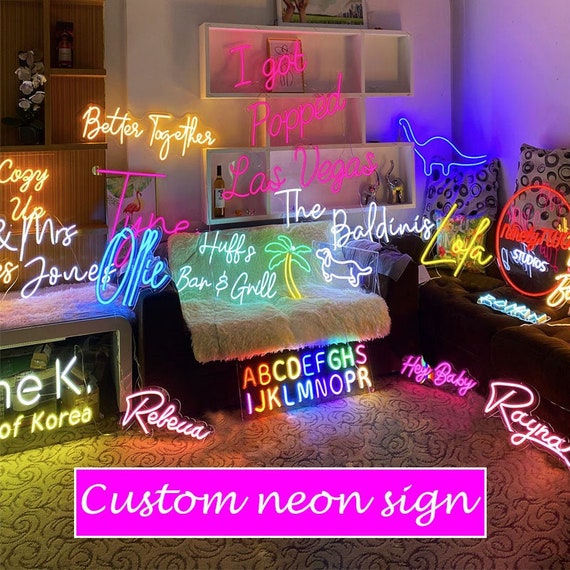This visually striking advertisement showcases a vibrant collection of custom neon signs arranged in a luxurious, eclectic room. The space is adorned with a floral-patterned carpet, fuzzy and decadent furniture, including brown and other colored sofas, as well as brown wooden pieces. Each neon sign is meticulously placed on various surfaces - from the floor to floating shelves on a white wall. The myriad of neon signs, totaling at least 15, displays a wide range of customizations, from business names like "Huff's Bar and Grill" and "Hey Baby Studios" to personal and whimsical sayings such as "I Got Popped Las Vegas," "Better Together," and "The Baldinis." The vibrant alphabet section showcases neon letters in a spectrum of colors, with a few letters appearing in primary hues. Situated at the bottom of the photo is a pink rectangular box with the words "Custom Neon Signs" elegantly written in white cursive, highlighting the service offered. The overall ambiance exudes creativity, encouraging viewers to imagine their bespoke neon creation.